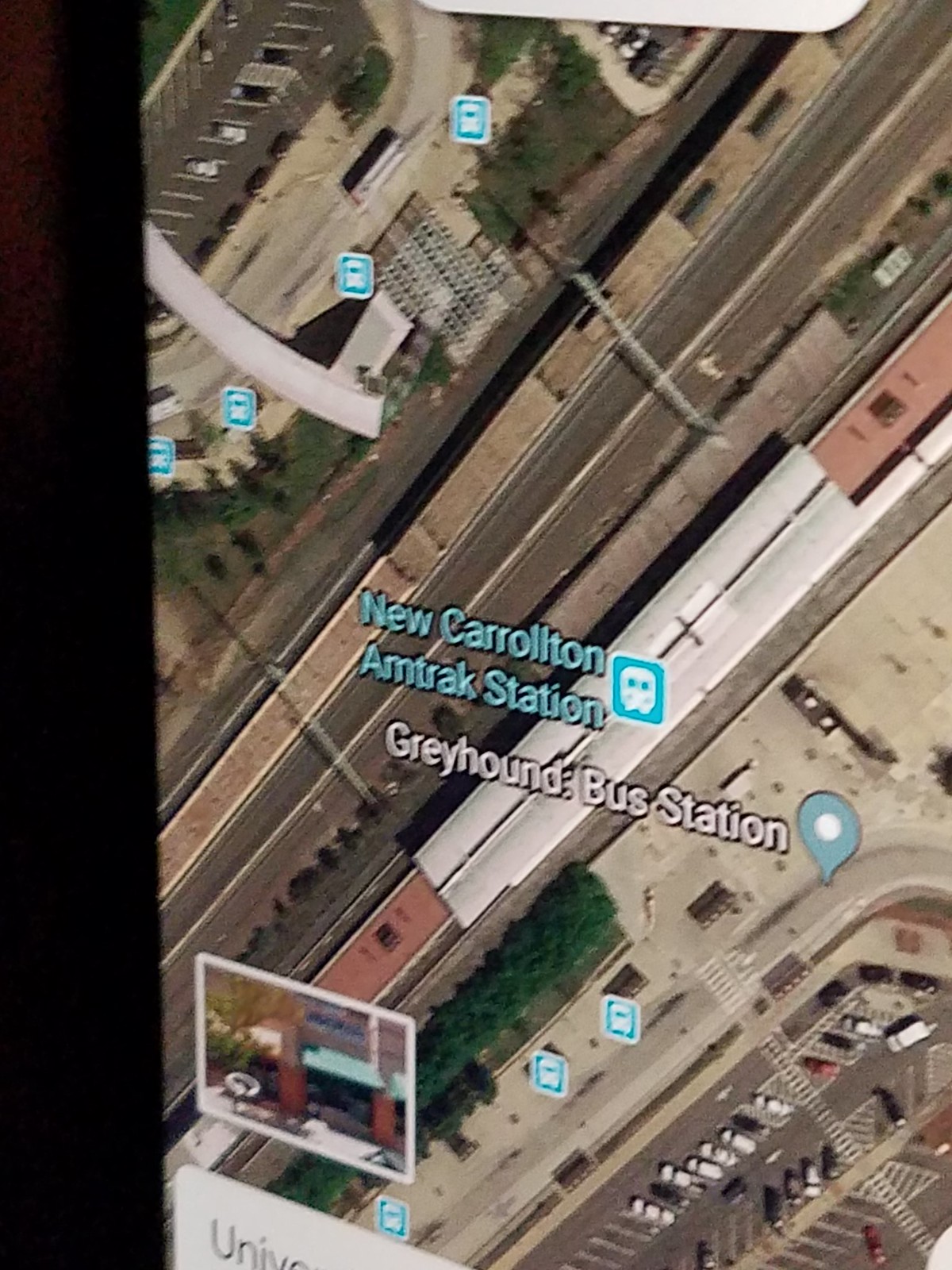The image captures a partially visible phone screen displaying an aerial view on Google Maps. The screen is clipped on the right, top, and bottom edges, cutting off parts of the display. The focal point is the New Carrollton Amtrak Station and the nearby Greyhound Bus Station, both labeled in distinctive text; the Amtrak station in turquoise and the Greyhound station in white. A prominent feature is a diagonal stretch of railroad tracks running from the lower left to the upper right, indicative of the transport hub's layout. The lower right section of the image features a detailed parking lot with three rows of angled parking spaces, while the upper left corner showcases another smaller lot with two rows of angled spaces. On the left side of the phone, the background is dark, hinting at a low-light environment. A small box in the bottom left of the phone screen offers a street view option, showing the building's front facade. Additionally, a white text box at the screen's bottom reads "Univ..." likely short for "University." The composition captures the busy, urban transportation nexus with clear, informative labeling and essential infrastructure elements.